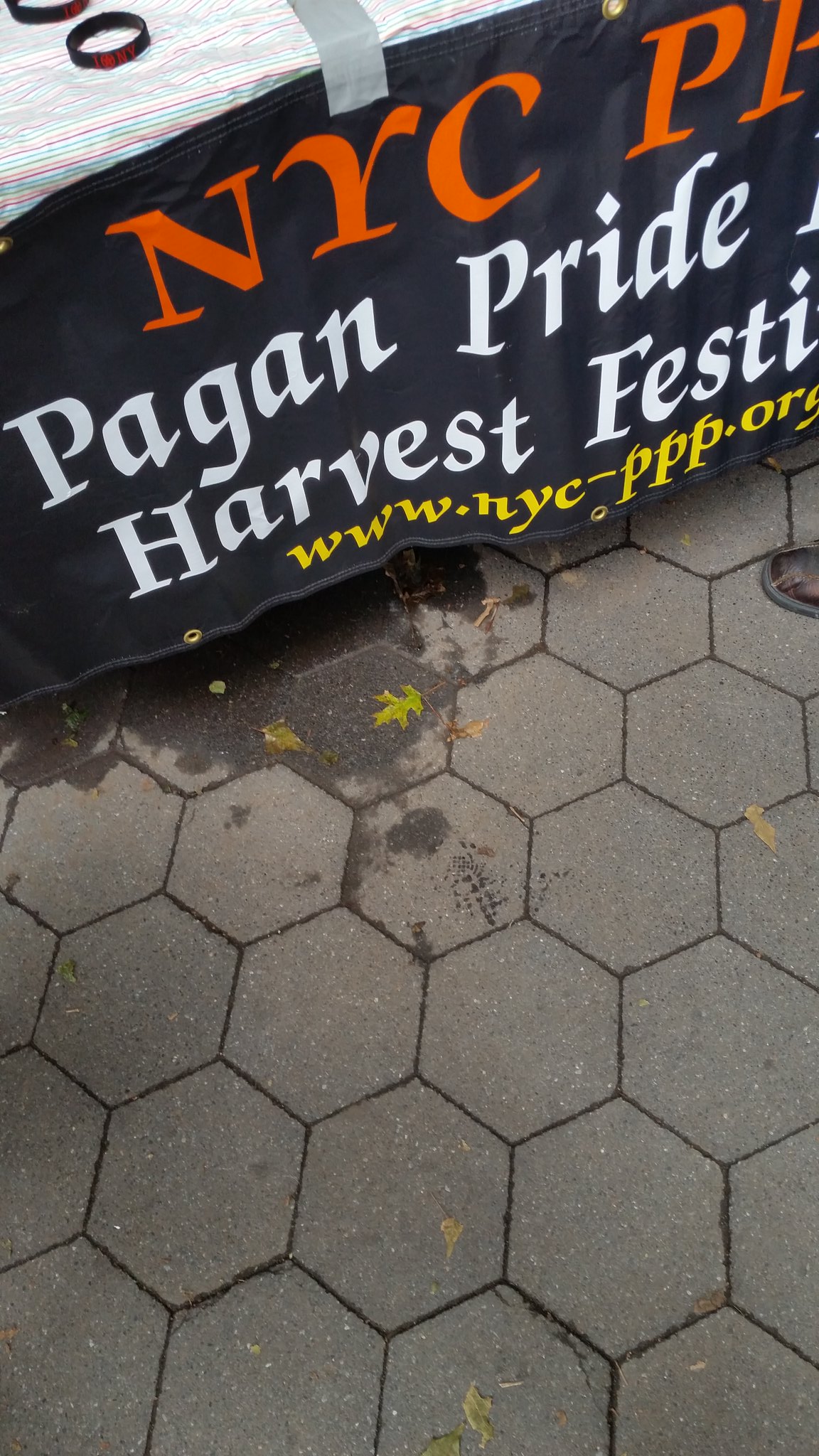The photograph captures an outdoor setting featuring a hexagon-patterned concrete sidewalk, some of which appears wet possibly due to recent rain, adorned with scattered leaves. In the foreground, there's a table draped with a vibrant, striped rainbow tablecloth. At the front of the table, a black banner, affixed with gray duct tape, prominently states "NYC Pagan Pride Harvest Festival" in bold colors—'NYC' in red, 'Pagan Pride' in white, 'Harvest Festival' partially visible also in white, and the URL "www.nyc-ppp.org" in yellow. On the table, amidst various free handouts, are black wristbands emblazoned with red "I Heart NY" text. The overall scene conveys a colorful and inviting atmosphere typical of a community event.